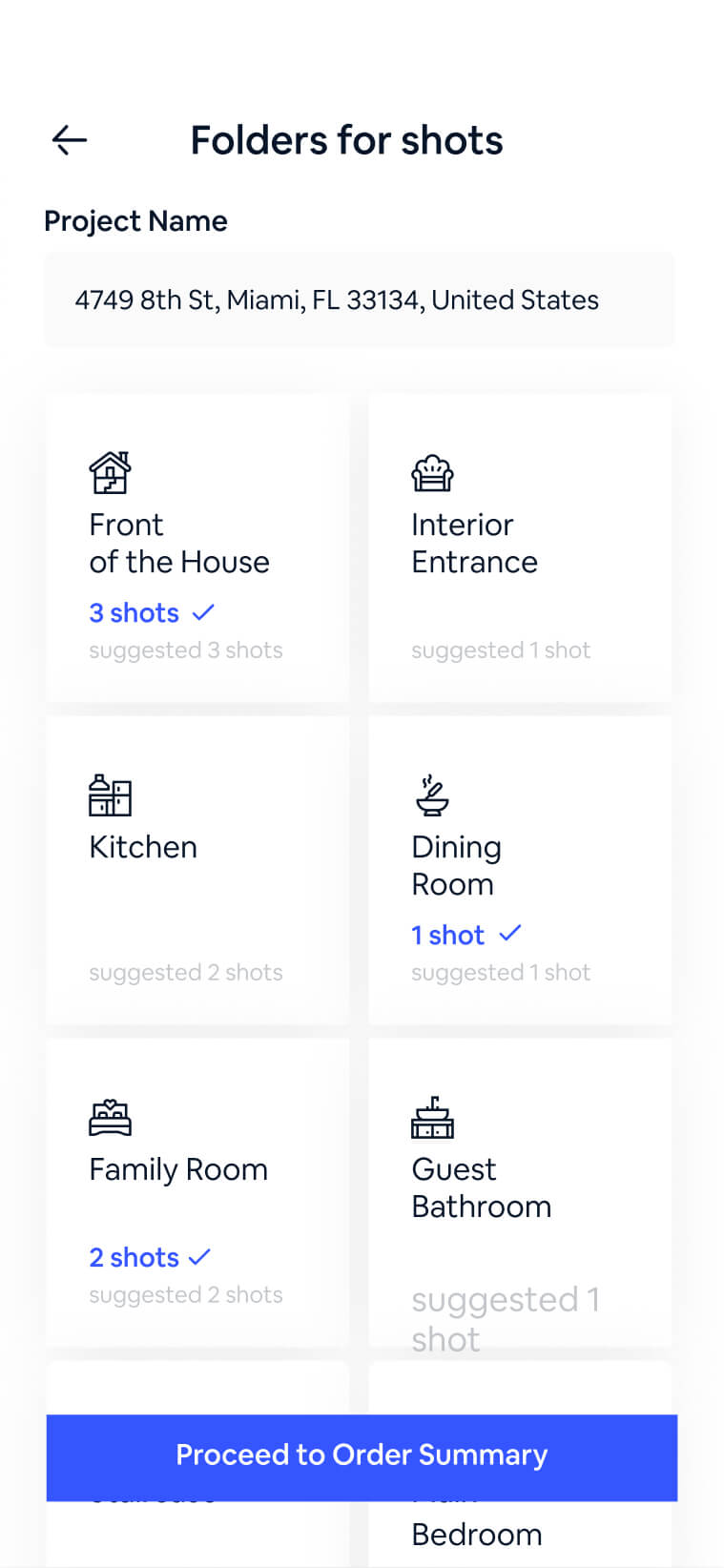The image showcases a detailed printout for a real estate photography project, titled "Project Name: 4749 8th Street, Miami, Florida, 33134, United States." The printout lists various categories of shots required for the property:

- **Front of the House:** Suggested three shots.
- **Kitchen:** Suggested two shots.
- **Family Room:** Suggested two shots.
- **Interior Entrance:** Suggested one shot.
- **Dining Room:** Suggested one shot.
- **Guest Bathroom:** Suggested one shot.

At the bottom of the document, the section labeled "Proceed to Order Summary" is highlighted in white. Directly beneath the word "Summary," the word "Bedroom" is printed in dark gray.

Each category with specified shot counts is highlighted in blue and marked with a checkmark, indicating the required images have been taken. Categories without completed shots lack this blue highlight and checkmark.

The printout also features corresponding icons for each chosen area:
- **Front House:** A house icon.
- **Interior Entrance:** Appears as a garage or similar structure.
- **Kitchen:** Depicted with appliance icons.

This printout appears to be part of a workflow for organizing and verifying real estate photography.